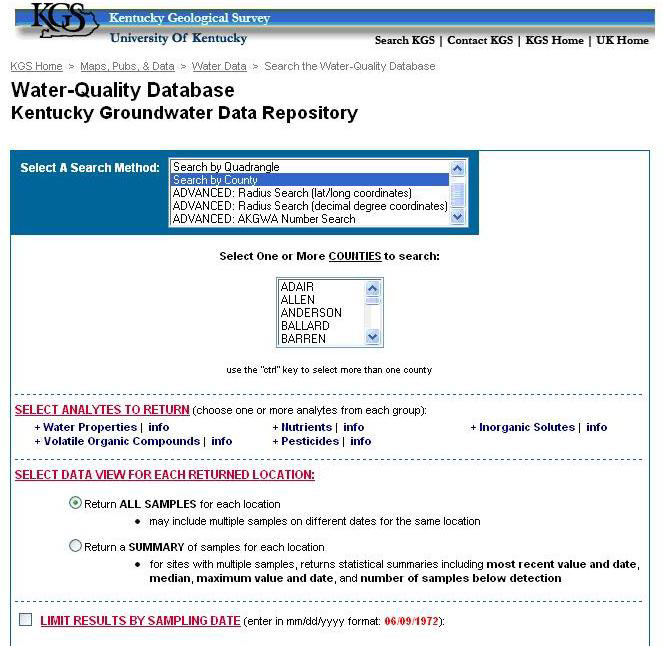**Detailed Caption:**

The image is a screenshot of the Kentucky Geological Survey (KGS) website. The top of the page features a small horizontal dark blue bar. On the left side of this bar, the logo "KGS" is displayed in black with an outline of Kentucky surrounding the letters 'S' and 'G'. To the right of the logo, the text "Kentucky Geological Survey" appears in white.

Below the blue bar, the background is white. Slightly to the right, the text "University of Kentucky" is written in dark blue. Further to the right are four clickable links in black text: "search KGS", "contact KGS", "KGS home", and "UK home".

Moving down to the left, there is a vertical column of menu options. The option "KGS home" is underlined in gray and has a right-facing arrow next to it. Following this, there is "maps, pubs, and data", also underlined in gray with a right-facing arrow beside it. Next, the option "water data" appears, also underlined in gray with a right-facing arrow. Lastly, "search the water quality database" is listed in gray text and underlined.

Underneath these options, the section heading "Water Quality Database Kentucky Groundwater Data Repository" is presented in bold black letters.

Continuing down, there is a blue outline box that encases a darker blue horizontal rectangle at the top left. Within this rectangle, the text "Select a Search Method" is displayed in light blue. To the right of this, there are several search options in black: "Search by Quadrangle", "Search by County", "Advanced Radius Search Latitude-Longitude Coordinates", "Advanced Radius Search Decimal Degree Coordinates", and "Advanced AKGWA Number Search".

In the middle of the page, centered, the instruction "Select one or more counties to search" is written in black, with the word "counties" underlined. Below this, there is a small drop-down box outlined in gray containing names of counties in black text. The visible names are "Adair", "Allen", "Anderson", "Ballard", and "Barron". Below the drop-down menu, an instructional note "Use the control key to select more than one county" appears in black.

Further down, there are two horizontal rectangles. The first rectangle is outlined with dots and has the text "Select Analytes to Return" in red at the top left. To its right, the message "Choose one or more analytes from each group" is written in black. Below these instructions, several categories are listed in black with "info" links next to each: "Water Properties", "Volatile Organic Compounds", "Nutrients", "Pesticides", and "Inorganic Solutes". Each category has a plus sign to the left for accessing a drop-down menu with additional options.